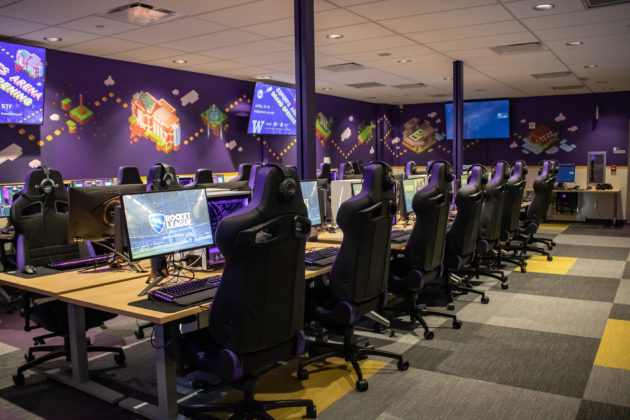This vibrant color photograph captures a cutting-edge gaming room designed for competitive gamers. Rows of high-performance computer setups, each featuring a monitor and keyboard, meticulously line the room. Flanking these setups, the walls are adorned with large electronic displays and monitors, each with its own queue of eager participants. The room is furnished with imposing black office chairs that boast high backs for comfort, each crowned with a pair of substantial black headphones.

The flooring features an eye-catching pattern of carpet tiles in shades of dark gray, light gray, and yellow, adding texture and depth to the space. The walls are painted a striking purple and embellished with dynamic orange and green decorations, evoking a vivid video game ambiance. Additional gaming stations are thoughtfully arranged along the walls, which are accented by light brown wainscoting that provides a subtle, sophisticated contrast. The room is completed with a clean, white suspended ceiling, further enhancing the bright and energetic atmosphere.